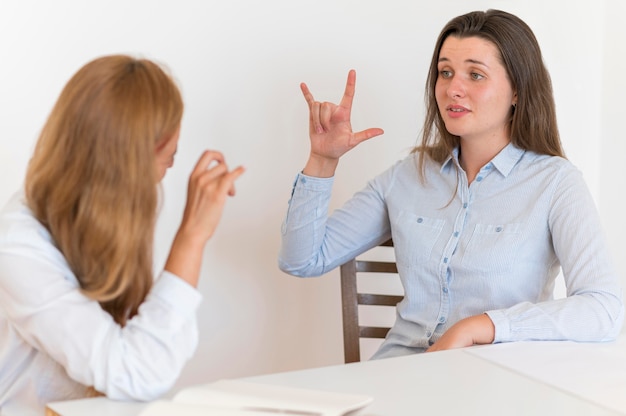In the image, two young women are seated at a white table, engaging in a conversation using sign language. The woman on the left has long reddish hair and is dressed in a white top. Her fingers are curved and wiggling as she communicates. Opposite her, the woman on the right has shoulder-length brunette hair and is wearing a light blue shirt with buttoned sleeves and pockets on each breast. She is making a sign with her right hand—two fingers up, two fingers down, and a thumb pointed out to the side. Both women appear to be deeply engaged in their conversation. The background features a white wall with a light source coming from the right, illuminating the setting. They are seated on wooden chairs, and there are pieces of white paper on the table in front of them.